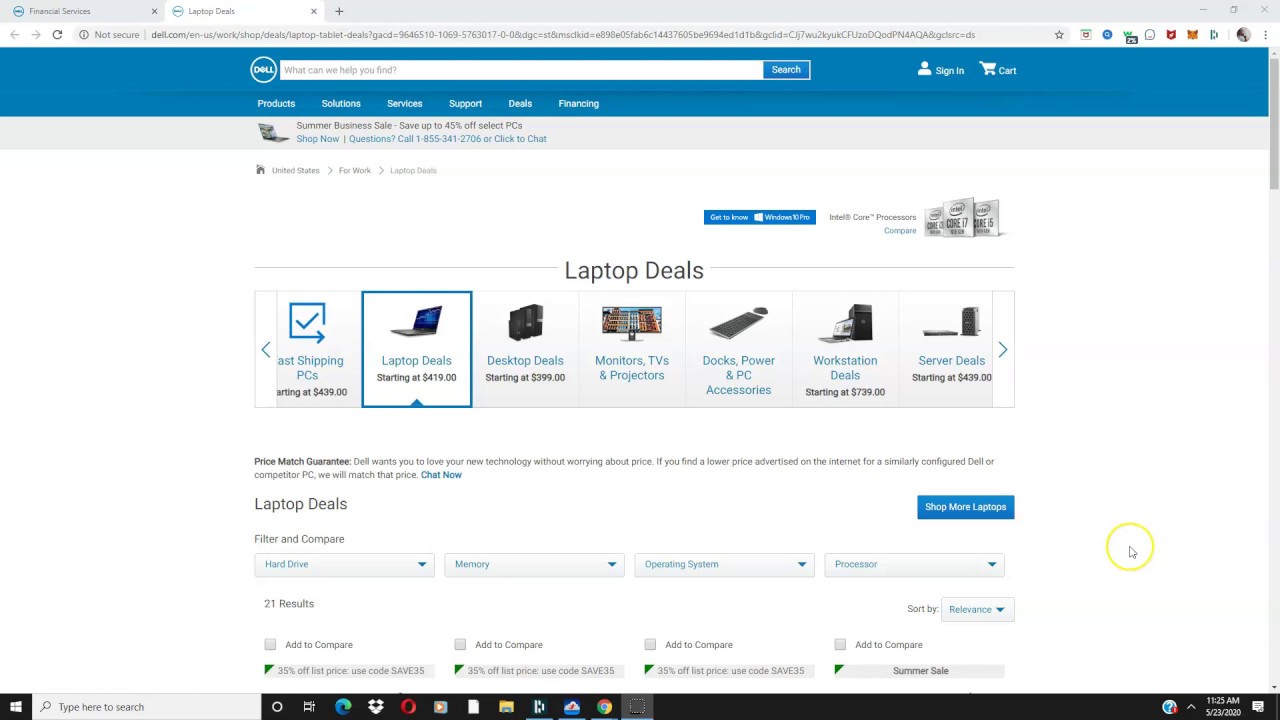This image, sourced from Dell.com, showcases a browser window focused on Dell's laptop deals. The browser has two tabs open, with the active tab being the one displaying the Dell laptop deals page, characterized by its white theme and blue Dell banner. Centrally placed is a circular Dell logo, featuring a white outline and text. Below the logo, a search bar with the placeholder "What can we help you find?" is accompanied by a blue search button. On the top right, a white person icon with a "Sign In" label can be seen next to a shopping cart icon labeled "Cart."

The navigation menu includes categories such as Products, Solutions, Services, Support, Deals, and Financing. Prominent in the display is a banner announcing a "Summer Business Sale" with savings of up to 45% off select PCs. The "Laptop Deals" section is highlighted, featuring various images of laptops. Additional categories include Desktop Deals with a tower icon, Monitors with a monitor icon, TVs & Projectors with a corresponding icon, Docks & Power Stations, Workstation Deals, and Server Deals. Each category is represented by an icon that visually describes the type of product offered.